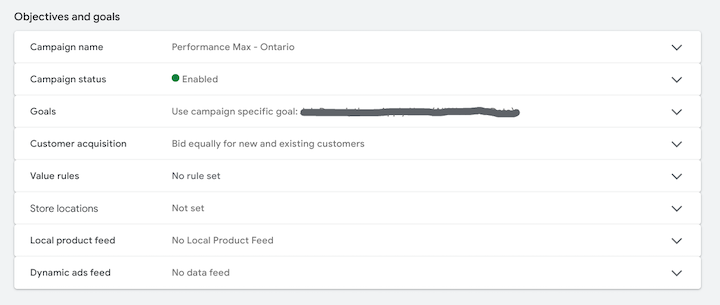This image displays a detailed "Objectives and Goals" section of a user interface, likely from a campaign management or analytics tool. The section consists of eight horizontal dropdown sections, each offering additional options when expanded.

In the top left corner, the title "Objectives and Goals" is prominently displayed in the darkest color text on the interface. The background of the overall section is a light gray, while the dropdown boxes themselves have a white background.

The first dropdown in the top left is labeled "Campaign Name" in slightly darker text. The currently selected campaign is "Performance Max Ontario." Adjacent to it, the box also provides options for later selections.

On the left side right below the campaign name, "Campaign Status" is indicated with the status as "Enabled," highlighted by a green button.

Further down, on the left, several other sections are listed:
- Goals: "Use Campaign Specific Goal," underlined by a horizontal gray line that spans most of the selection.
- Customer Acquisition: Specified for “Equally for New and Existing Customers.”
- Value Rules: Currently set to "No Rules Set."
- Store Location: Shows "Not Set."
- Local Product Feed: Indicates "No Local Product Feed."
- Dynamic Ads Feed: Displays "No Data Feed."

Although the "Goals" section has an emphasis with a large gray horizontal line, it appears uneven and shaky, resembling an annotation made using a paint tool.

This detailed interface is functional for users aiming to manage and customize campaign objectives efficiently. The structured yet descriptive elements make each section easy to identify and interact with for different campaign-related settings.